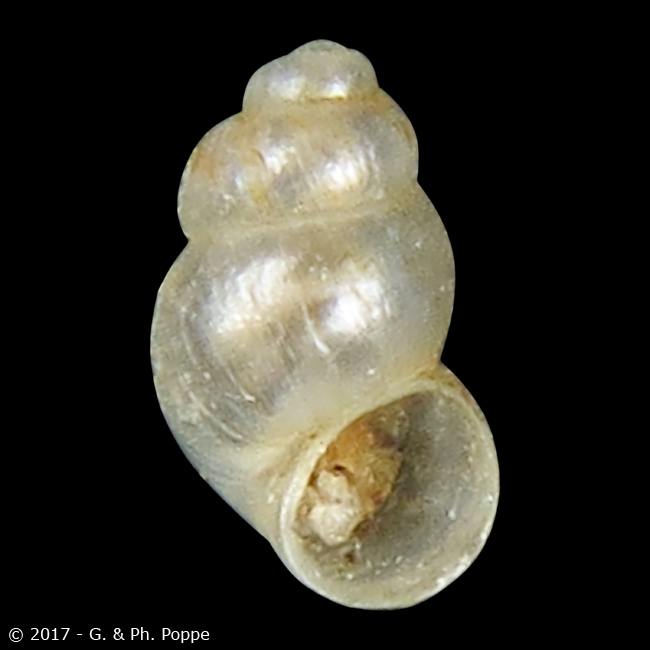This image features a carefully composed close-up photograph of an upright, translucent shell from some form of mollusk, possibly a snail or a sea snail. The shell, pearl white in color, stands against a stark, detail-free black background which accentuates its smooth, polished surface. Light from above creates reflections on the shell, highlighting its opaque yet transparent qualities. Inside the shell, there appears to be remnants of dried, organic material, suggesting the previous presence of a mollusk, adding a layer of historical intrigue to the artifact. The photo is marked with a copyright symbol and the text "2017-G & P.H. Pope," located at the bottom left corner, indicating ownership by the photographer Pope.